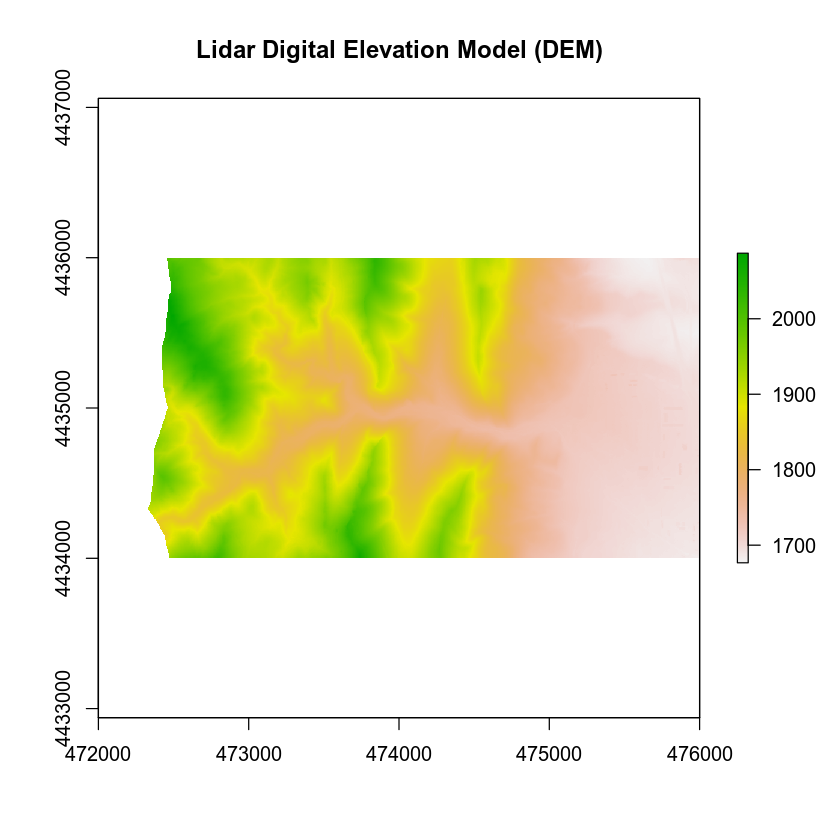The image is a LiDAR Digital Elevation Model (DEM) showcasing a detailed topographical representation. The elevation is color-coded, transitioning from green to yellow to orange to red, as indicated by the key on the right, which ranges from 1700 to 2000. The x-axis spans from 472000 to 476000, while the y-axis extends from 4433000 to 4437000. Most of the left side of the image features green and yellow hues, indicating lower elevations, gradually transitioning to pink on the right side for higher elevations. The model is centered on the graph, with large numerical labels marking the bounds on both axes.